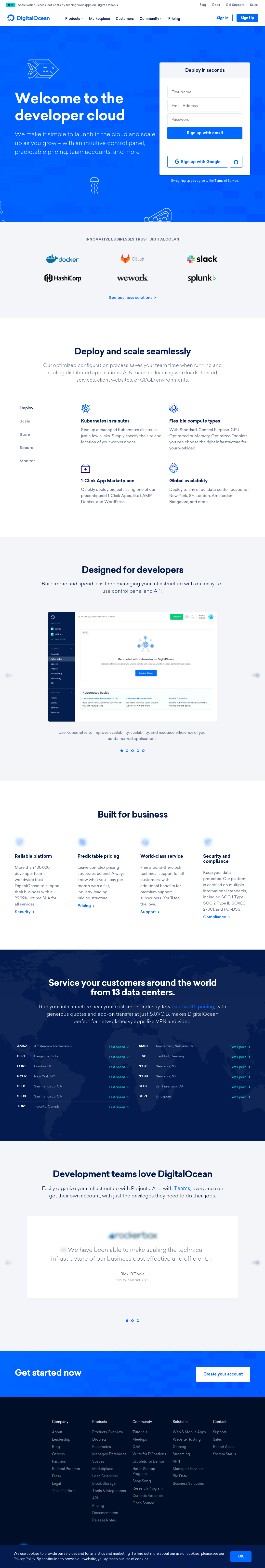This image showcases the full layout of a website, likely intended for desktop use given the amount of detail visible. The layout is vertically compressed, displaying the entire website at once.

The top section features a navigation menu, followed by a large blue banner that states, "Welcome to the Developer Cloud," with sign-in options positioned to the right. Beneath this banner, a series of logos including those of Slack, WeWork, and Splunk, among others, are displayed to indicate partnerships or services.

The next section carries the tagline, "Deploy and Scale Seamlessly," and introduces a sidebar menu on the left with five navigational options. On the right, there are four highlighted areas in bold text, probably describing key services or features available.

Further down, a section titled "Designed for Developers" appears, which seems to showcase an admin page relevant to the services offered. This is followed by another segment, "Built for Business," which includes four paragraphs, each accompanied by headers and small icons, likely explaining various business-oriented features.

A prominent blue field with a stylized planet background follows, containing the text, "Service your customers around the world from 13 data centers." Below this, another section promotes Digital Ocean with the phrase, "Develop Teams Love Digital Ocean," and a call-to-action field for getting started, presented in another blue box with an input field for user interaction.

The layout concludes with a large footer that includes comprehensive contact information and other essential links.